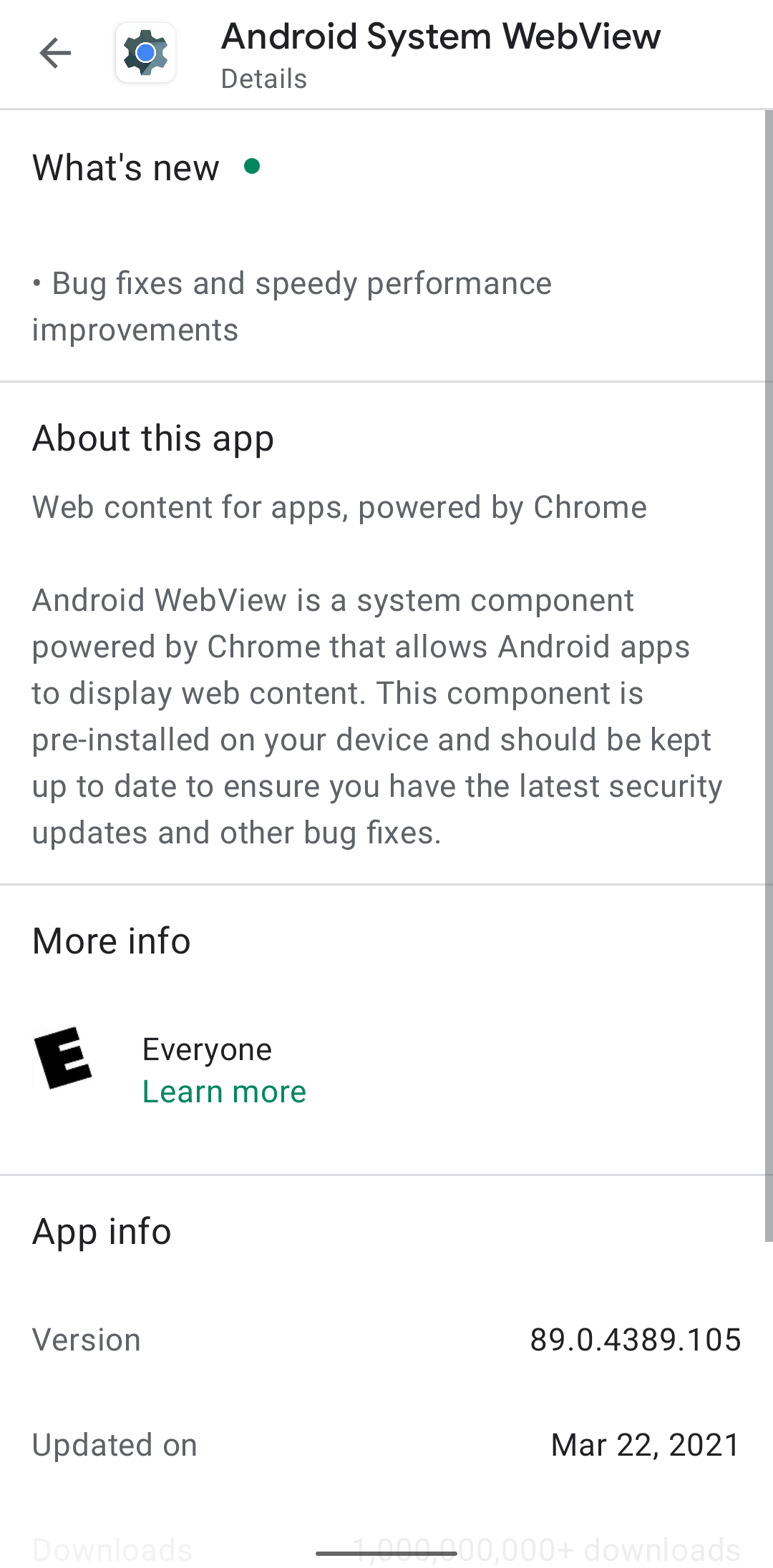The image showcases a white phone screen displaying detailed information about the "Android System WebView" app. 

At the top-left corner, there is a back arrow icon followed by the settings app icon. To the right of these icons, the text "Android System WebView" is prominently displayed. Below this, in smaller font, additional details about the app are provided. A horizontal line spans the screen beneath these details.

Below the line, a section titled “What’s New” appears with a green dot next to "New". Following this is a bullet point reading, "Bug fixes and speedy performance improvements."

Another horizontal line separates this section from the next, which is labeled "About this app". This section describes the app in detail: "Web content for apps, powered by Chrome. Android System WebView is a system component powered by Chrome that allows Android apps to display web content. This component is pre-installed on your device and should be kept up to date. Here, you have the latest security updates and other bug fixes."

Following this explanatory text, yet another horizontal line is displayed. Below this line, the text "More info" is present, accompanied by a black "E" icon and the word "Everyone". In green text beneath this, it says "Learn more".

Another line continues across the screen, under which resides the section titled "App info". Here, "Version" is listed on the left side as "89.0.4389.105" and "Updated on" with the date "March 22, 2021".